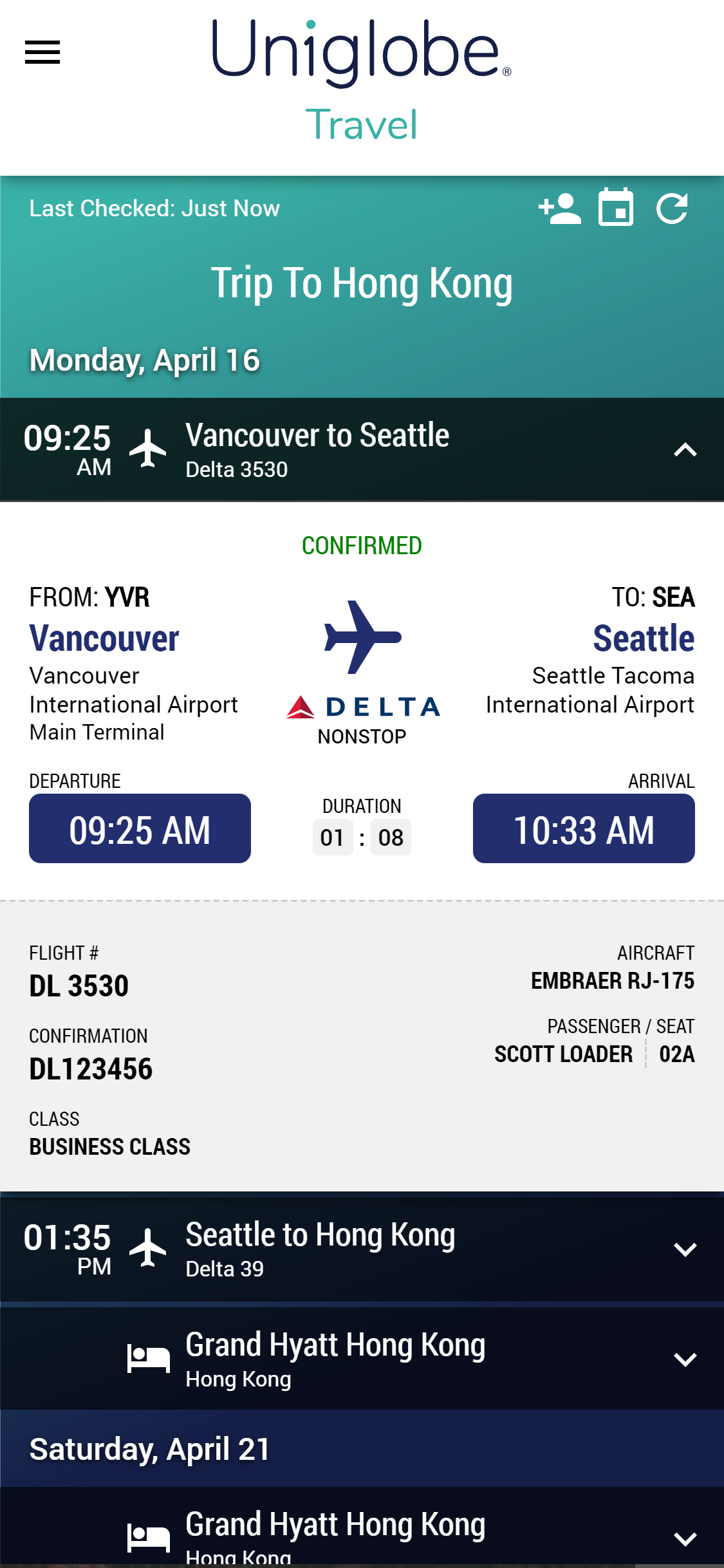A detailed itinerary screenshot from the Uniglobe Travel mobile app, featuring a travel plan for a trip to Hong Kong last checked just now. The journey commences on Monday, April 16th, with the first leg being a flight from Vancouver to Seattle. This segment is operated by Delta Air Lines, Flight DL3530. The flight departs from Vancouver International Airport (YVR), specifically from the main terminal, at 9:25 AM and is scheduled to land at Seattle-Tacoma International Airport (SEA) at 10:33 AM. The duration of the flight is 1 hour and 8 minutes. The confirmed flight details include the flight number DL3530 and the confirmation code DL123456. The traveler, Scott Loader, will be flying in business class on an Embraer RJ175 aircraft and is assigned to seat 02A.